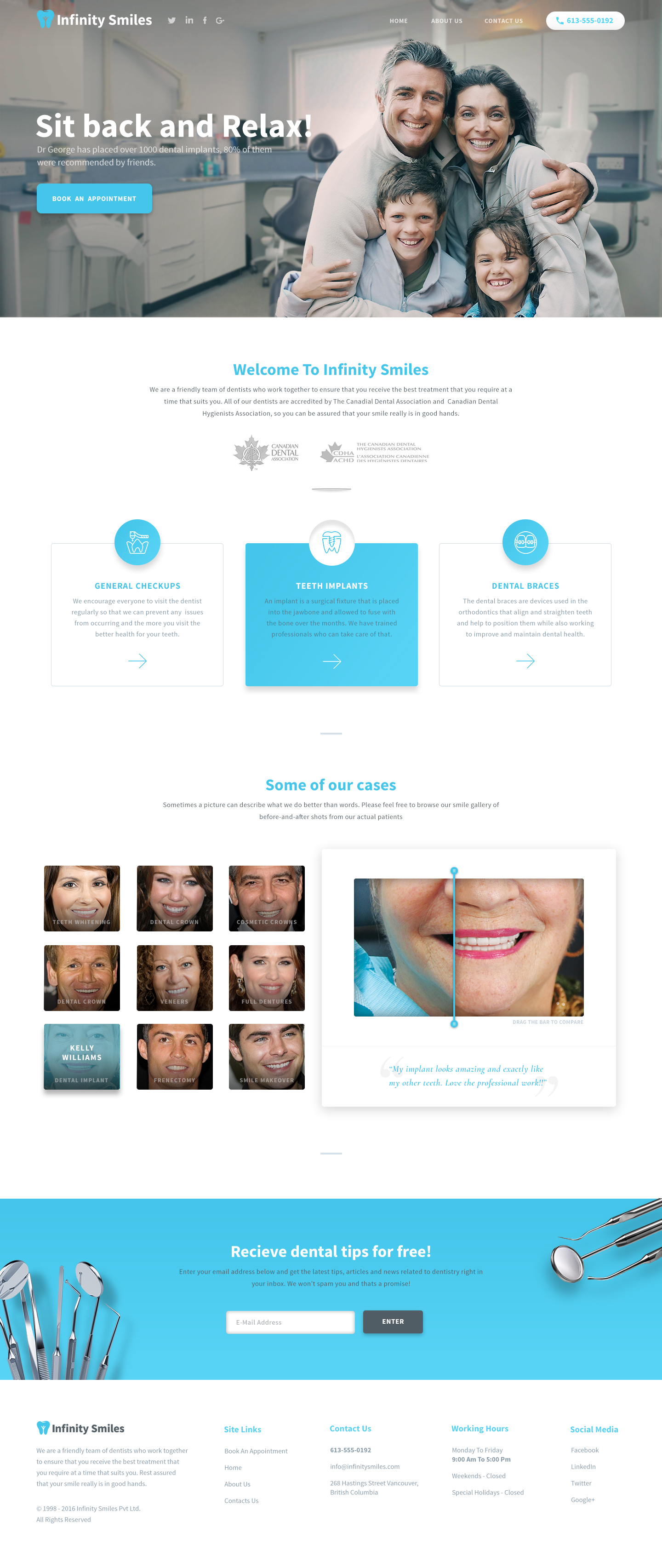The screenshot captures a vertically oriented web page for "Infinity Smiles," prominently displaying a blue logo featuring a tooth on the left side. There are social media icons for platforms such as Twitter, Instagram, Facebook, and Google. At the top of the page, a navigation bar includes links to "Home," "About Us," and "Contact Us," along with their phone number enclosed in a blue circle.

The background image showcases a traditional family—a mother, father, and two children (one boy and one girl)—all wearing beige and gray quarter-zip clothing. They are smiling and posing in front of a dentist's office, evidenced by visible dental equipment and a dental chair. 

Below this, there is a blue box inviting users to book an appointment. This section is followed by an informative area discussing Infinity Smiles, detailing services offered such as general checkups, teeth implants, and dental braces. Next, the page highlights various celebrities purported to be patients, showcasing treatments they have received like veneers, dental crowns, cosmetic crowns, full dentures, and teeth whitening.

Further down, there's a segment offering free dental tips, adorned with dental equipment imagery. The bottom of the screenshot includes additional site links for easy navigation.